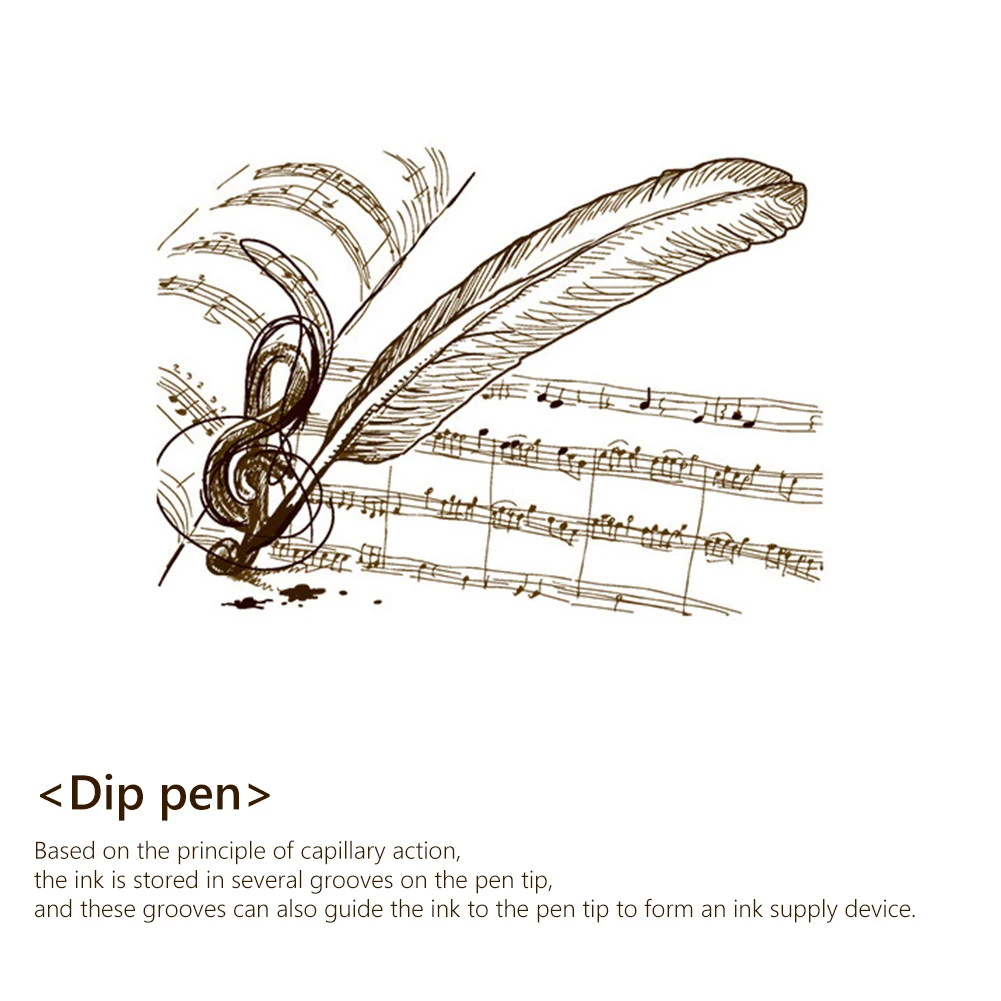The image depicts a detailed pencil drawing of an open music sheet spanning two pages. On the left page, there are six lines of handwritten music notes, featuring a prominent treble clef and suggesting a fairly fast tempo. The right page, slightly turned, shows four lines of music notes from the middle downward. At the bottom left corner of the right page, a three-dimensional, dark black music note is illustrated, with a black-and-white feather plume attached to it, simulating an old-fashioned dip pen. The pen, based on the principle of capillary action, stores ink in several grooves on the pen tip, allowing the ink to flow smoothly when writing. Bold black lettering at the bottom of the image reads “dip pen,” accompanied by smaller text explaining the ink storage mechanism and functionality. The overall focus is on the dip pen and its historical ink distribution method, integrated with the creative process of music notation.